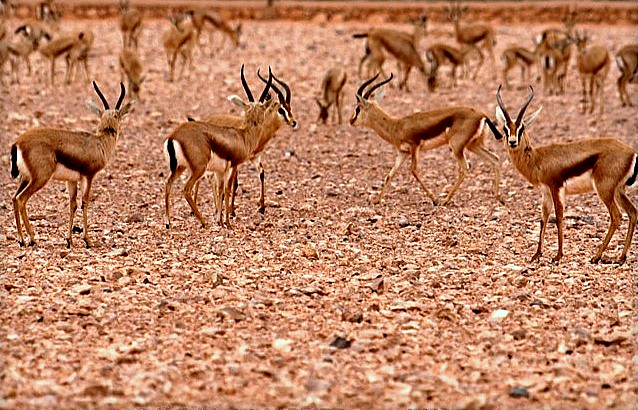The image features a detailed, side-view close-up of a natural setting. The ground is a light brown, covered with what appears to be a mix of mulch, small rocks, and pebbles of various colors, including white, black, brown, and gray. Scattered throughout this earthy terrain is a herd of slender, four-legged animals resembling antelopes or deer. These animals have brown backs, white stomachs, and distinctive black tails. Their long, V-shaped antlers or horns, which curve at the tips, extend elegantly from their heads. A prominent feature is the striking pattern around their faces: black fur behind the eyes outlined with white fur, creating a vivid contrast. Some of these creatures have their heads down, while others face the camera, with their big white ears clearly visible. In the slightly blurred background, more of these antelopes can be seen, continuing the scene of this natural tableau.